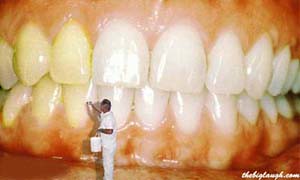The image depicts what appears to be an advertisement for teeth whitening, featuring an artistic installation of a gigantic mouth. The close-up view showcases both the upper and lower sets of teeth, emphasizing the gums and teeth with dramatic detail. A tiny man, dressed entirely in white and carrying a white bucket, stands just to the left of the center near the area of the canine teeth. He appears to be painting the teeth white; the teeth immediately to his right are noticeably whiter and cleaner, while the teeth to his left remain yellow and discolored. The gums beneath the yellow teeth are bleeding, whereas the gums beneath the whiter teeth have just a slight hint of blood. The man’s face, turned away and blurry, features dark hair, obscuring his facial details. There's an unreadable signature or text located at the bottom right corner of the image, adding an element of mystery to this striking and surreal composition.